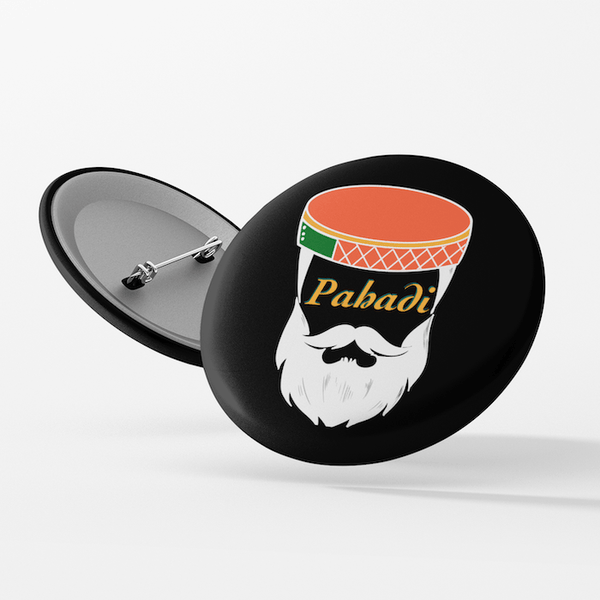This detailed image shows a pin against a grayish-white background. The left side of the frame features the back of the pin, highlighting its silvery horizontal needle and matte light gray finish, all encircled in black. The right side displays the front of the pin, characterized by a matte black background. The pin showcases a silhouetted black face adorned with a white beard and mustache, which have dark gray vertical highlights and are outlined in black. Across the face area in vivid orange text, the word "Pahadi" is inscribed. Atop the head, there's a salmon-orange flat cap, featuring a green rectangle on the left and an orange rectangle with white X’s on the right, separated by a yellow band at the top.